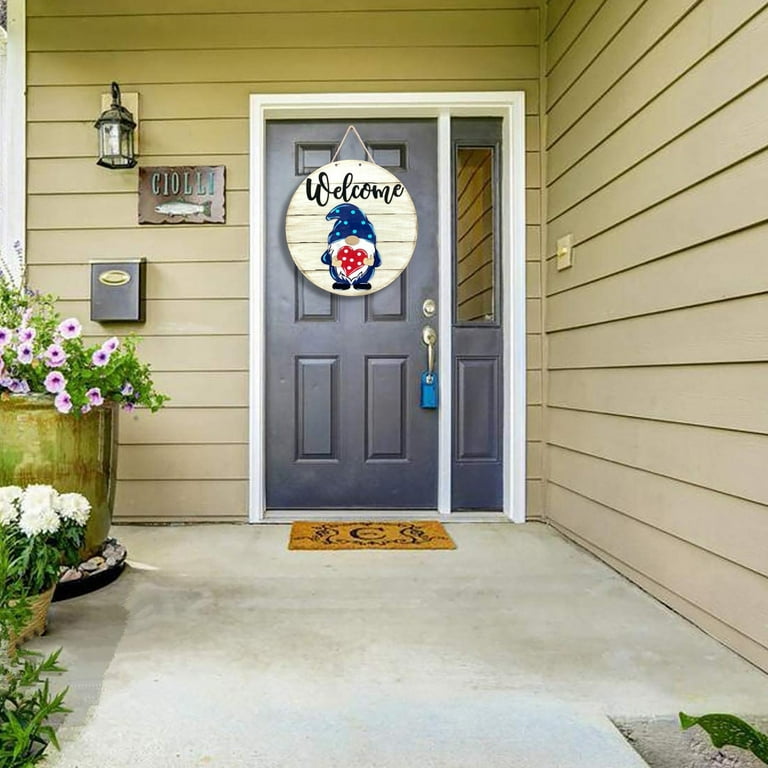This image captures the inviting front of a beige house with horizontal wood siding. At its center is a dark gray door adorned with a wooden circular welcome sign that features a gnome holding a polka-dotted red heart and wearing a blue hat with light blue dots. Flanking the door is a vertical window section separated by a white 2x4. To the left of the door, a family name plaque that reads "YALI" sits above a fish symbol, along with an old-fashioned hanging lantern and a small letterbox. Below the door lies a welcome mat on a gray concrete area, with the boundary of the concrete visible in the bottom right. Potted plants, including a large golden pot with pink, purple, and white flowers, and a smaller brown bronze pot with white flowers, add a touch of nature near the doorway. Additionally, a realtor lockbox hangs from the door's bronze lock, indicating the house may be on the market.